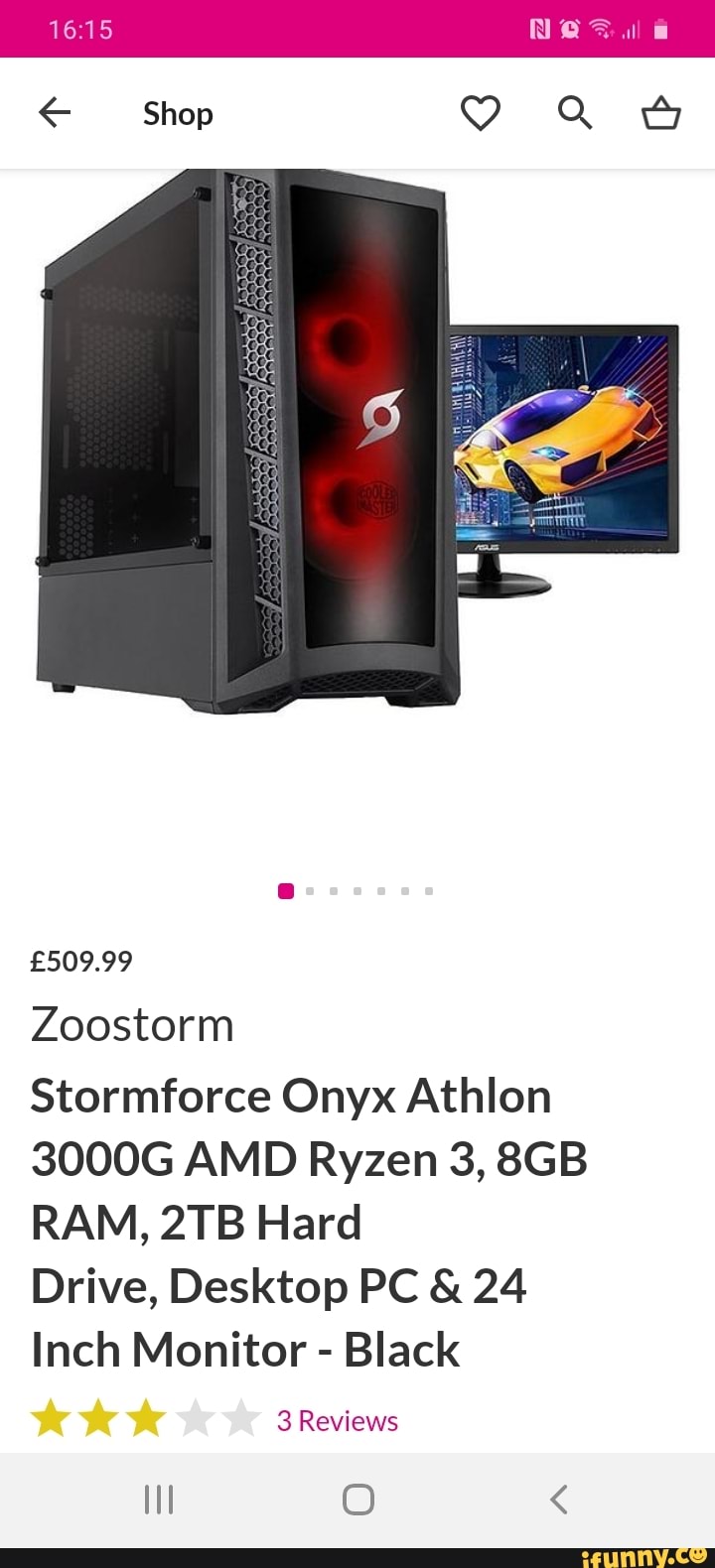Screenshot of a shopping platform at 4:15 p.m., displaying a product page for a "ZooStorm StormForce Onyx Athlon 3000G AMD Ryzen 3 Desktop PC with 8GB RAM and 2TB Hard Drive, including a 24-inch Monitor in black." The mobile device showing the screenshot has approximately 85% battery, strong cell service, and Wi-Fi connection. The top toolbar, colored pink, features several icons including an alarm, cell strength, Wi-Fi indicator, and battery charge. Below, a white taskbar features a back button, the shop's logo, a heart icon to favorite the product, a magnifying glass for search, and a basket icon for the cart. The product is priced at £509.99 and has a three-star review. The image displays both the desktop tower and the monitor.